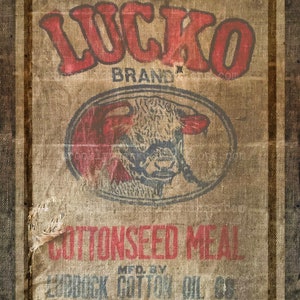This image captures a vintage-style package labeled "LUCKO Brand Cotton Seed Meal." The central text features "LUCKO" and "Cotton Seed Meal" prominently in bright red, while the word "Brand" is subtly in black. Below this, additional black text states, "MFD by Lubbock Cotton Oil Co." The label, appearing to be distressed paper, exhibits a worn, brownish hue and is framed by a darker brown border. A line-drawn cow logo, accented in black and red, adds a rustic charm to the package, hinting at its agricultural roots and historical significance.